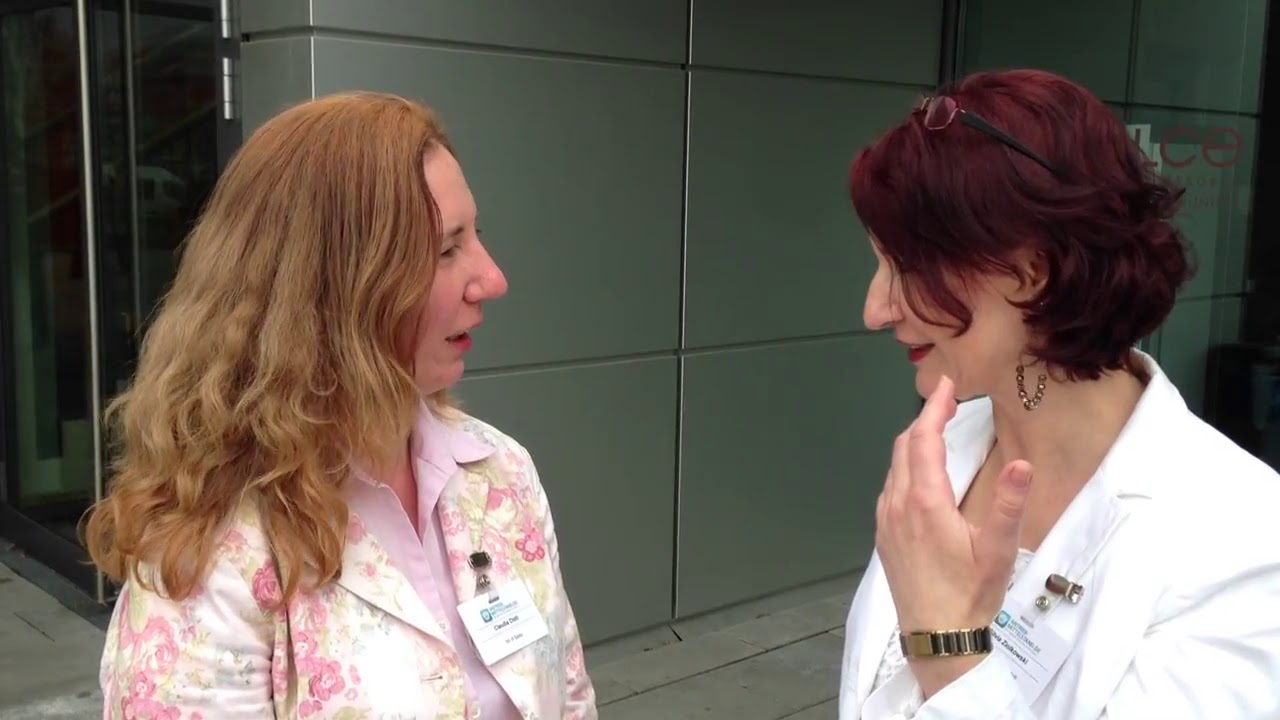In this detailed image, two female doctors are engaged in a deep conversation outside a green-walled building. Positioned center-frame, the woman on the left has striking red hair and is dressed in a light floral jacket over a pink collared shirt, her name tag placed above her left breast. She is animatedly speaking to the other woman, who has dyed dark red hair and wears a white doctor’s coat with a white shirt underneath. Notably, this second woman has a bracelet on her left wrist, gold earrings, a pair of glasses resting atop her head, and a name badge above her left breast. The backdrop features glass doors flanking both sides and some windows adorned with logos. The scene is set on what appears to be concrete steps or flooring, illuminated by daylight, showcasing an outdoor professional interaction.